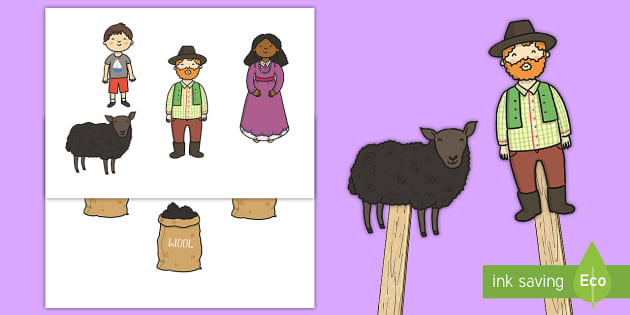This horizontally aligned rectangular image showcases a lavender-purple background with no borders. On the left, there is a white square section depicting animated characters: a black sheep with a gray hood, a boy in orange shorts and a gray t-shirt, a man donning a brown hat, brown pants, and a green shirt, and a woman with dark skin, black hair, and a long purple dress. Overlapping this, a second white square displays three sacks, with one clearly visible brown sack labeled "wool" in white letters, containing black material. On the right side of the image, against the purple background, are Popsicle sticks - one with an image of the previously mentioned sheep and another with the man in the brown hat and pants. The lower right corner features text against a green rectangular backdrop, reading "Ink Saving" in white letters, accompanied by a water droplet or leaf symbol, and the word "eco."